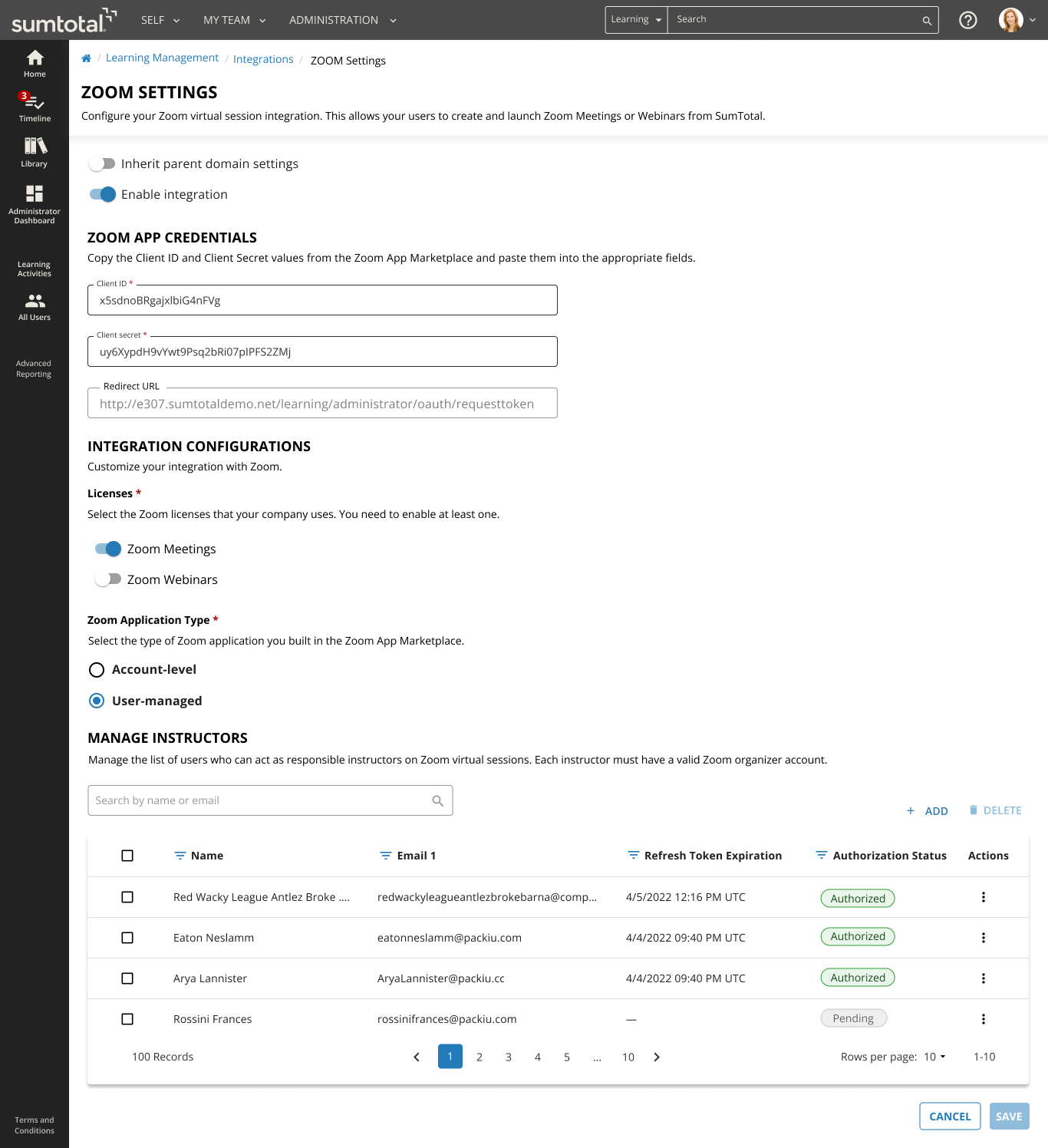The image is a screenshot of a landing page for configuring Zoom settings, possibly integrated within a management platform called "SumTotal." In the top left corner, there's a label that says "SumTotal." Below this, aligned to the left, are various icons including a home symbol, a timeframe icon, a summary/library icon, and additional unidentified symbols.

On the opposite side, towards the top right, the heading reads "Zoom Settings: Configure your Zoom virtual session integration." The page description underneath explains that it allows users to create and launch Zoom meetings and webinars directly from the SumTotal platform.

At the bottom-right part of the screenshot, there are two buttons labeled "Cancel" and "Save." Directly beneath the "Zoom Settings" section is a segment labeled "Credentials," where the user can enable Zoom integration. It is specified that the configuration options are available for Zoom meetings, with the Zoom application type set to "User Managed."

Finally, at the very bottom of the screenshot, there's a configuration section for managing users on the page. The entire interface is designed to streamline the integration of Zoom meetings and webinars within the SumTotal environment.